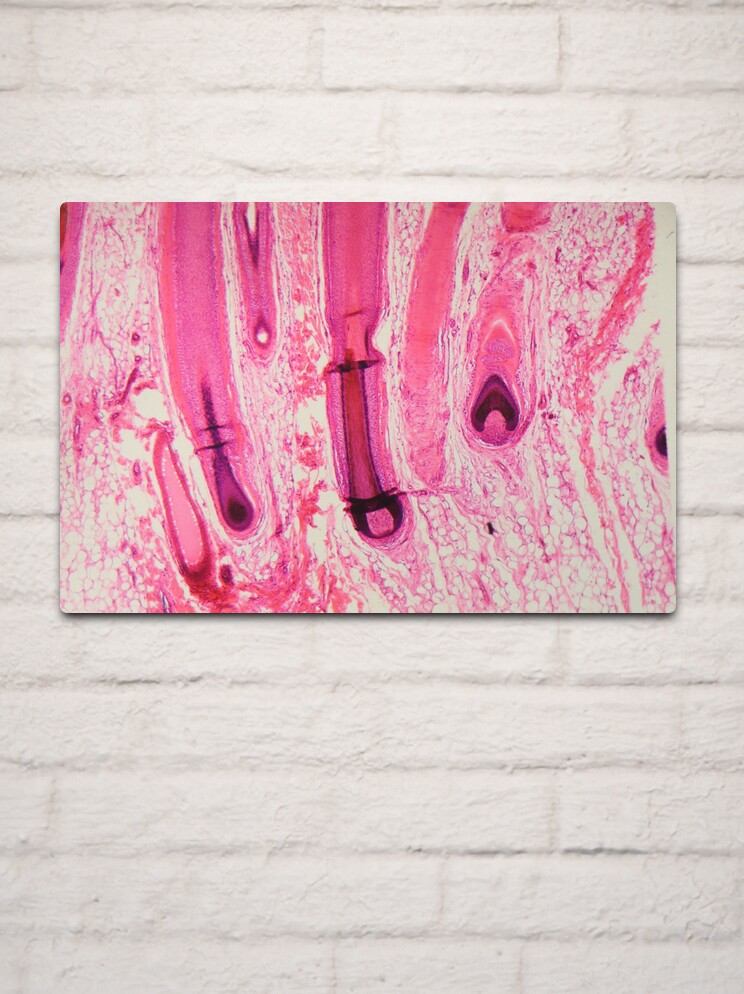This image features a detailed, abstract painting placed against a white-painted brick wall. The rectangular canvas, made from a beige material, prominently showcases bold, tubular strokes and splashes of varying shades of pink—ranging from light pink to dark magenta—and occasional dark purple accents. These strokes, which form elongated, oval shapes, evoke a microscopic view of human tissue, possibly depicting fibrous muscles and cells. The artwork lacks any textual elements or artist's signature, emphasizing its abstract and interpretative nature. White spots and paint intermix with the dense pink and purple strokes, creating a layered, complex composition that stands open to personal interpretation.